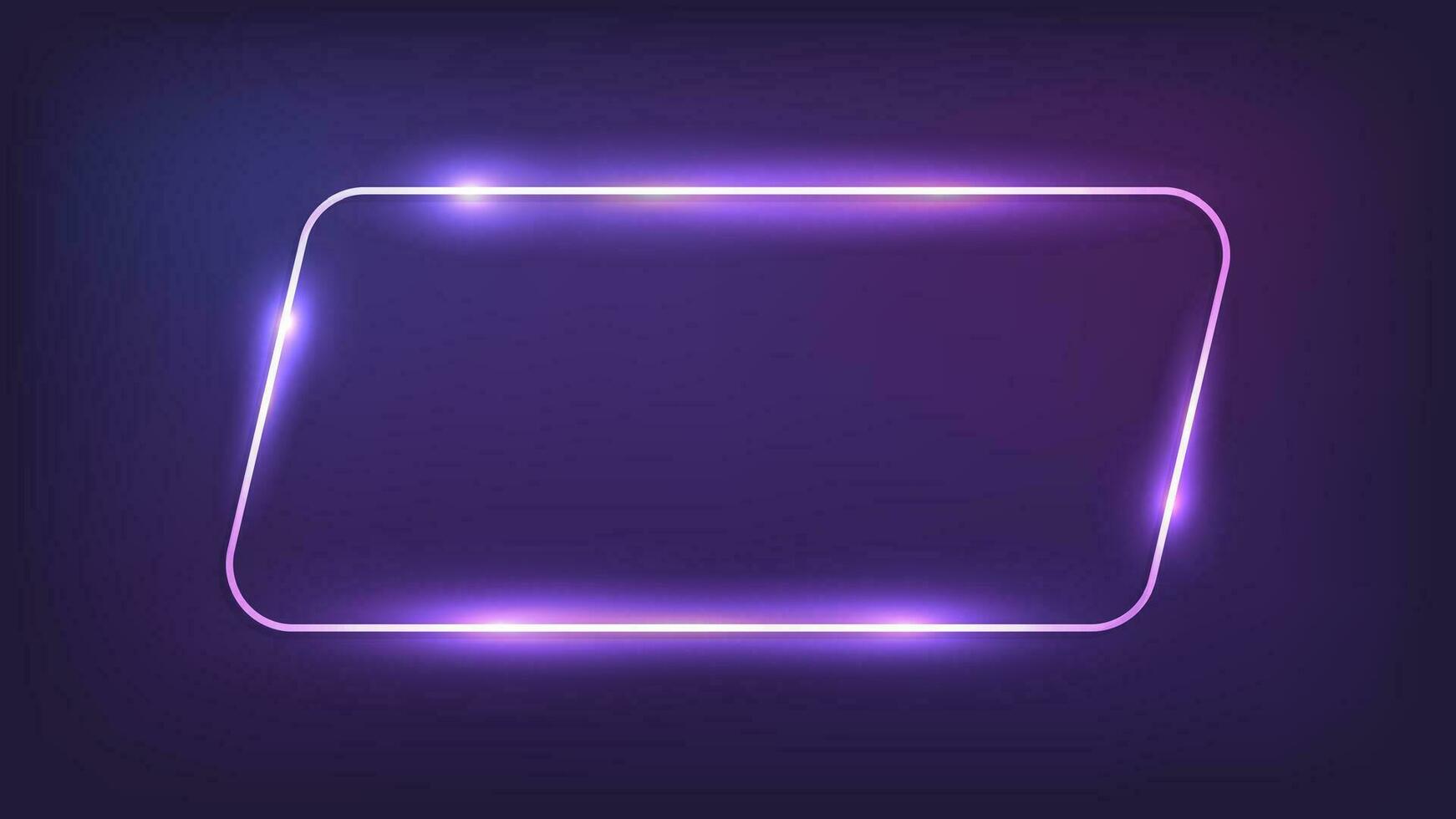The image features a prominently centered, rounded trapezoid (or rhombus) that occupies about 75% of the frame, set against a dark, deep purple background with a gradient that darkens towards the edges. The shape itself is outlined by a single silver line that glows with a pink and white gradient, creating a neon-like, tubular appearance. The illumination is most intense along the centers of each side rather than uniformly distributed, giving off a sporadic and dynamic glow. The interior of the shape and its surrounding background are a grayish-black color, reinforcing the dramatic lighting that spans the edges of the trapezoid. The overall effect is reminiscent of a light-up mouse pad or a digitally generated logo design, exuding a futuristic and sleek aesthetic.